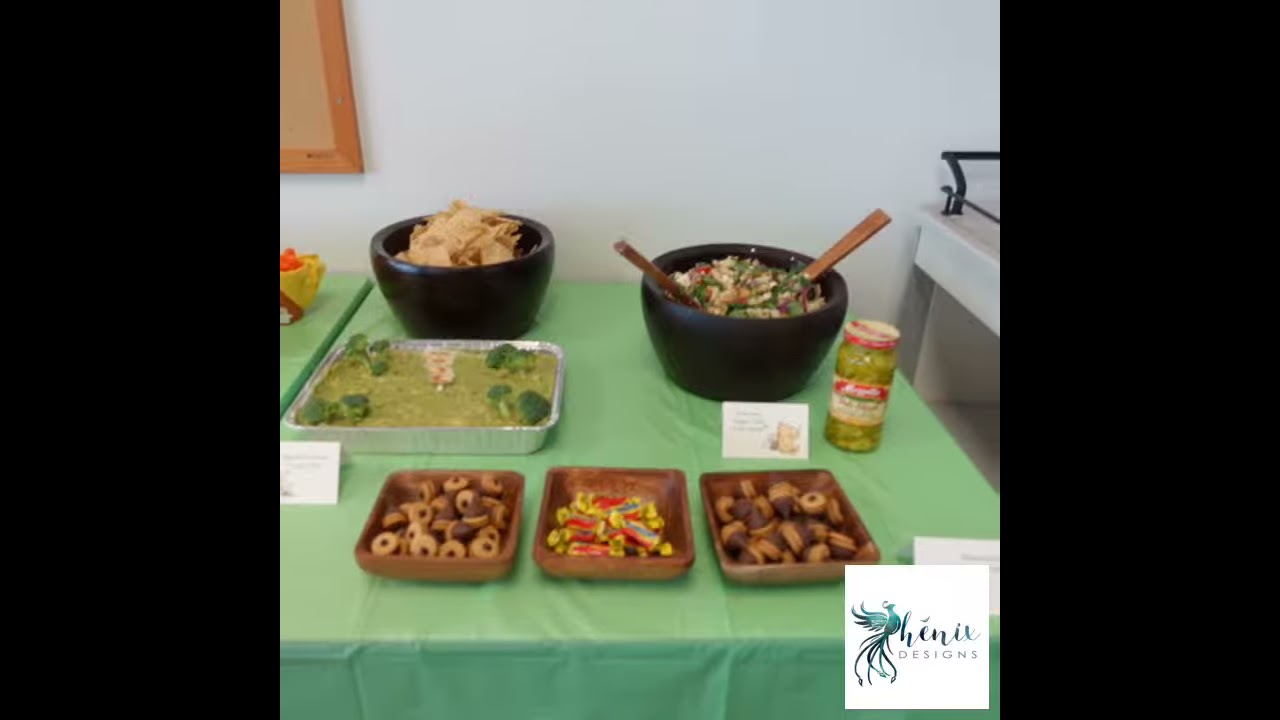The image displays a table adorned with a light green, possibly sage-colored plastic tablecloth, set against a white wall. At the back of the table are two large, black bowls. The bowl on the left is filled with nacho chips, while the one on the right contains a pasta salad, equipped with wooden spatulas or spoons and accompanied by a jar of peppers. To the left of the black bowls, there's another smaller black bowl containing salsa or a small salad.

Moving towards the foreground, there is a metal tray holding a green avocado dip with broccoli florets inserted into it. In front of this tray and closer to the viewer are three wooden square bowls. The first wooden bowl likely contains assorted small cookies, the middle bowl holds candies wrapped in red and yellow paper, and the third bowl also holds some cookies or possibly nuts.

At the very bottom right corner of the image, the logo “Fenny Designs” is visible, with the "P" stylized as a blue peacock.